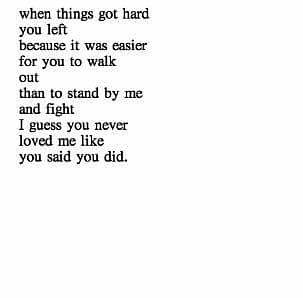The image showcases a poignant, text-based poem on a white background with black text. The poem is formatted into ten separate lines, all written in lowercase. Each line is consistent in style, giving the appearance of an excerpt from a book or a carefully constructed piece of poetry. The lines read:

"When things got hard,
you left,
because it was easier
for you to walk
out
than to stand by me
and fight.
I guess you never
loved me like
you said you did."

The text seems to have some subtle shadowing, possibly from the age of the image or the scanning process. The poem conveys a deep sense of sadness and heartbreak, likely reflecting a personal experience of the author. Its raw and simple presentation underscores the emotional weight of the words, which many might find resonate with their own experiences of love and loss.